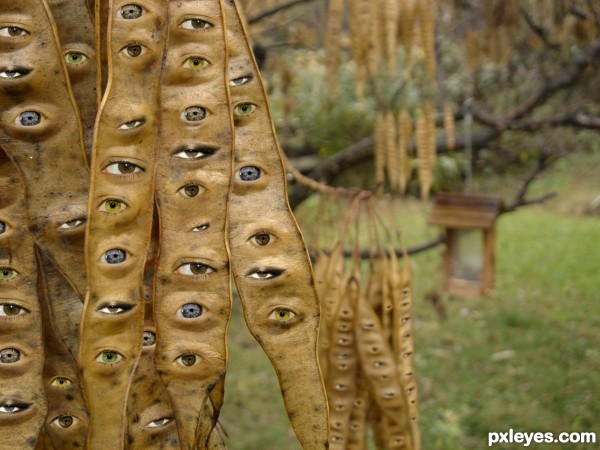This computer-generated image, possibly AI-created, shows an eerie and surreal scene of a tree with several long, flat, tan-colored seed pods that resemble dried brown or green beans. These seed pods, visible on the left side and scattered throughout the image, are vertically covered with human or animal-like eyes in various colors—blue, yellow, and brown. Each pod has a column of six to eight eyes, giving an unsettling effect. The background is blurred, revealing more tree branches adorned with these eye-covered pods, and a grassy area stretching beneath. A small wooden structure with a roof and two side supports can be seen in the middle right third of the image. The bottom right corner features the text "PXLEYES.com" in white.